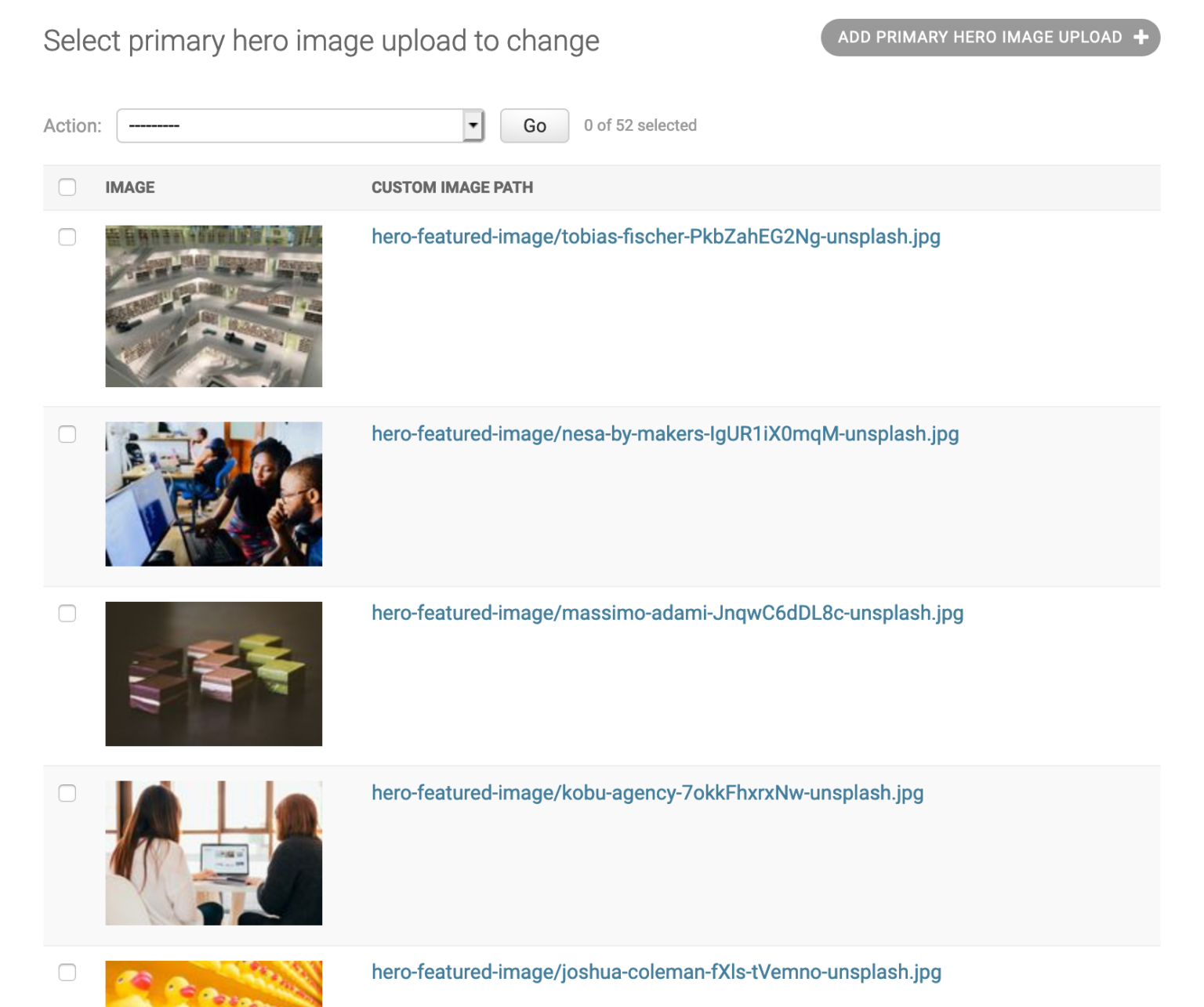The screenshot depicts a user interface for selecting and uploading hero images. On the left, there are several checkboxes for image selection, all currently unchecked. At the top left, the label "Action:" appears in small, light gray font, followed by a dropdown menu with a white background and gray outline. Adjacent to the dropdown are several gray dashes and a 3D-style gray button labeled "Go" in black text.

Above this section is a header in gray text reading, "Select Primary Hero Image Upload to Change." To the right, a medium gray, oval-shaped button features the text "ADD PRIMARY HERO IMAGE UPLOAD" in white, capital letters, accompanied by a bold cross icon.

Beneath this, a light gray header bar offers a "Select All" checkbox on the left and the word "IMAGE" in small, bold, gray, uppercase letters. On the right, a similar font indicates "CUSTOM IMAGE PATH." Below the header, a list of several images is displayed:

1. An aerial view of a city or several buildings.
2. A group of friends looking at computer screens.
3. An assortment of dark maroon, light brown, and green boxes.
4. Two women viewing a computer screen.
5. Rows of rubber ducks, although this image is partially cut off about one third down the page.